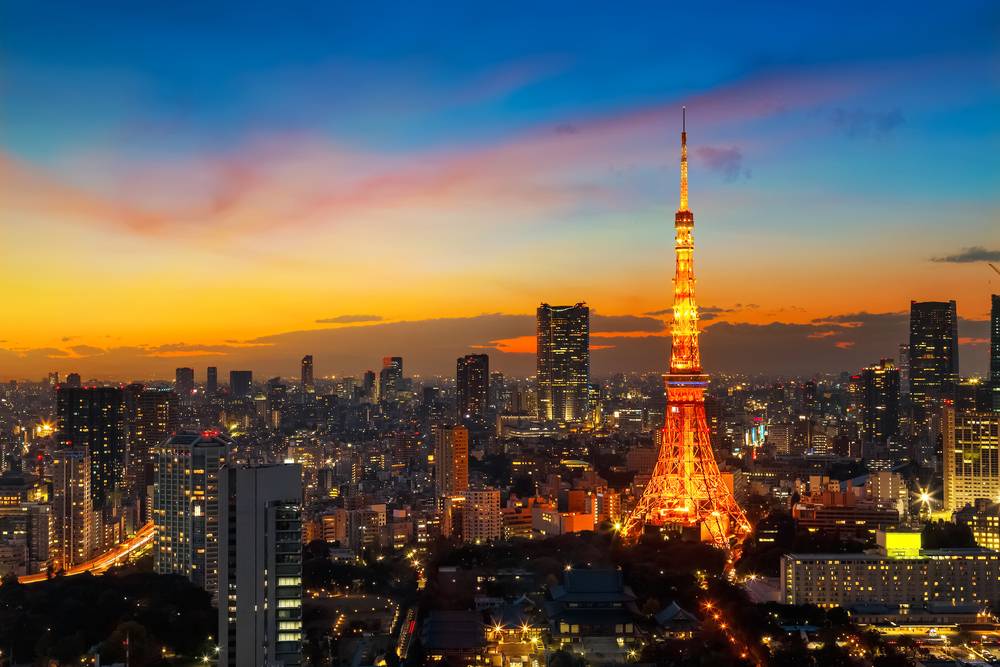An aerial view of Paris at dusk reveals the dazzling Eiffel Tower, brilliantly lit in gold, white, and orange hues, standing prominently in the right foreground. This iconic landmark is the brightest part of the scene, surrounded by an array of buildings of various heights, from 10-story structures to soaring skyscrapers. The city extends outward, dotted with street lights and illuminated windows, creating a vibrant mosaic of red and yellow lights from the traffic below. The sky above transitions beautifully from a dark blue at the top, through shades of light blue, to deep orange and yellow near the horizon where the sun is setting. Clouds in the higher atmosphere reflect a reddish tint, adding depth to the twilight spectacle. A large screen is visible to the right of the Eiffel Tower, contributing to the urban landscape. The nearby park is dark, with trees casting silhouettes against the twilight sky, enhancing the serene yet bustling ambience of the Parisian evening.